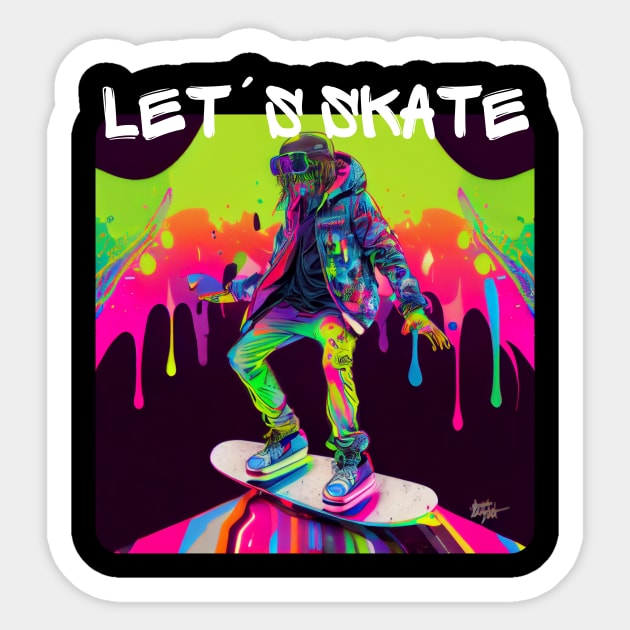This is an image of a skateboarder set against a vibrant, colorful backdrop. The image is framed by a layered border with a white outer frame and a black inner frame. At the top, overlapping the black border, there's text in white font that reads "Let's Skate." The skateboarder, mistaken for a snowboarder due to their attire, is skating over a flat, wave-like surface, rich with dripping paint in hues of pink, green, yellow, turquoise, and blue. The skateboard is white on top and beige in color. The skateboarder is clad in ski goggles that obscure their eyes, with long hair covering much of their face. They are wearing a blue jacket and shoes that match the colorful theme of the background, which overall gives the image a vibrant and dynamic feel. The paint drips and the detailed use of color enhance the energy and motion of the scene, creating a visually striking effect.